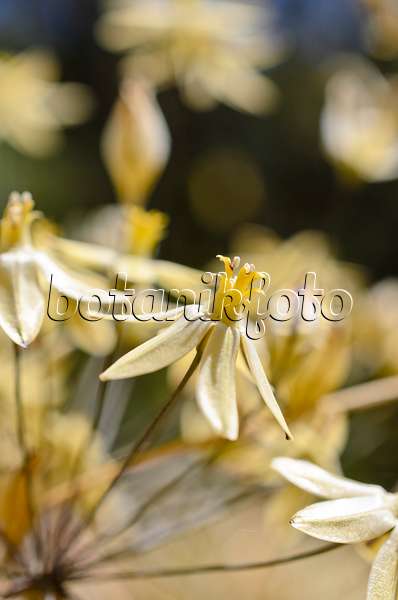The image captures a close-up of a pale yellow flower with drooping petals and a prominent central bud. The flower stands out in sharp focus against a backdrop of blurred, similarly colored flowers and green foliage. The background includes varying shades of green and hints of brown, creating a natural, scenic contrast. The centered flower features five delicate petals that curve downward, resembling bananas, and are attached to a brown stem. The overall effect is both serene and striking, enhanced by the blurred depth-of-field. Across the middle of the image, a watermark reads "botanikfoto" in lowercase letters, indicating either the creator or an ad for a botanical photography brand.